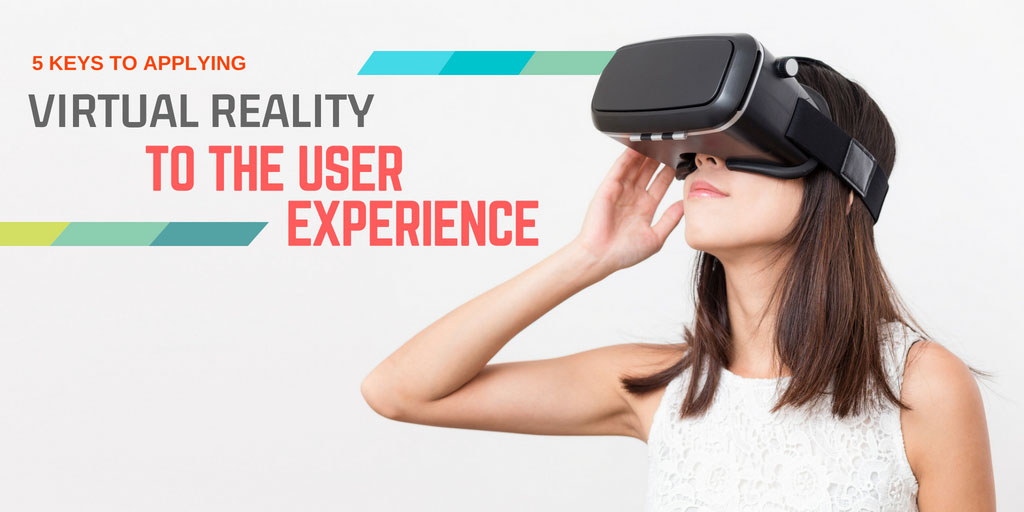A Caucasian woman with shoulder-length brown hair and wearing a sleeveless white lace top is engaged with a virtual reality instrument, holding the black VR headset on her head with her right hand. She has an upward glance and a slight smile, clearly captivated by what's happening inside the headset. Positioned on the right side of the image, she is juxtaposed with an advertisement on the left. The advertisement features the heading “Five Keys to Applying Virtual Reality to the User Experience.” The text, displayed in a combination of black and bold red letters, is accompanied by decorative green, blue, and turquoise bands designed to catch the eye. The background is a pale white, providing a clean contrast to the vibrant colors and highlighting the instructional nature of the content.